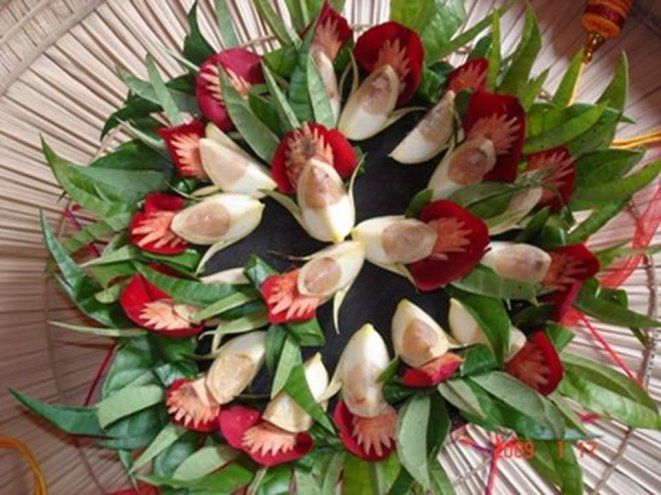This is an aerial perspective photograph featuring a meticulously arranged circular pattern of leaves and flower petals, atop a textured white paper surface with spiral-like creases resembling spokes radiating from the center. The outer ring of the composition features primarily green leaves, meticulously arranged to form a dense green perimeter. Moving inward, a striking array of flower petals showcases white and red hues, where the red petals have a distinctive peach-colored center. Some petals have been described as having an appearance similar to quartered eggs, with white and pink sections. Additionally, a smooth black surface is visible beneath the arrangement, adding contrast to the layout. Small strands of red and yellow ribbon or twine are also visible around the corners of the image, adding subtle accents to the composition. Overall, the intricate details and colors create a visually engaging floral design.